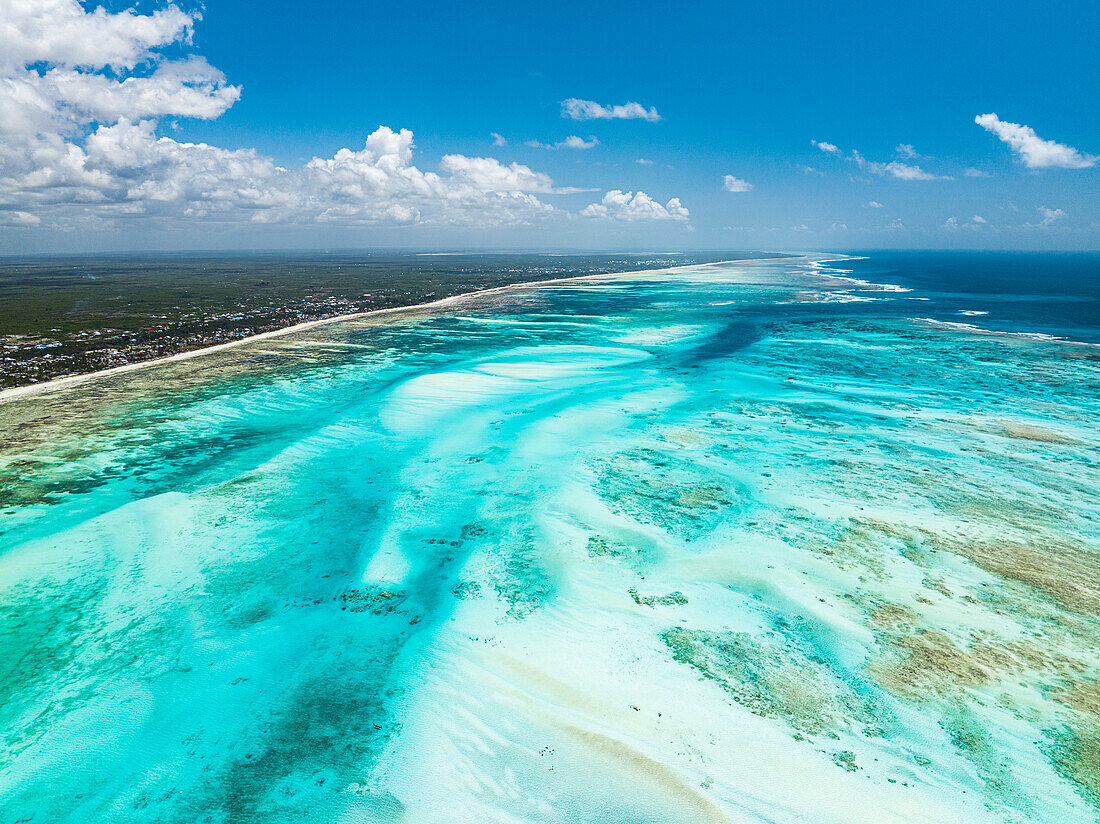This aerial photograph showcases a stunning coastline characterized by a blend of natural colors and elements. The scene features bright blue shallow waters extending along a wide shoal, bordered by pristine white and golden sand beaches. Further inland, you can observe a strip of green land, followed by a line of tan or beige terrain that appears to be washing into the ocean. In the upper right-hand quadrant, the dark blue waters of the open ocean meet the intricate patterns of white foam and waves crashing onto the shore. Beyond the beach, a road lined with houses and a small town stretches towards the horizon on the left side of the image. The sky above is a vast expanse of blue, punctuated by a large bank of clouds drifting in from the left and a few thinner clouds scattered throughout. This vibrant and serene summer scene captures the essence of a coastal paradise with its vivid hues of blue, green, and tan, and the subtle blend of human habitation and untouched nature.